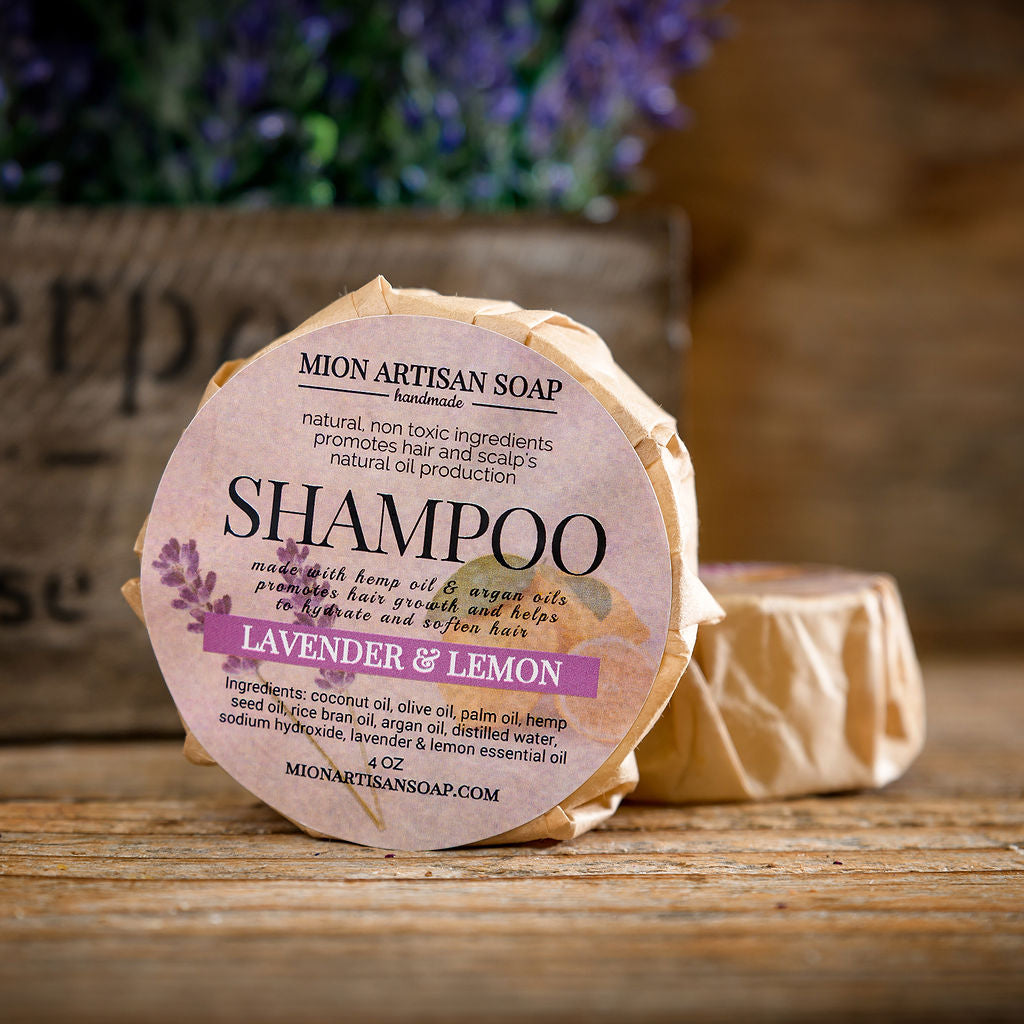The image showcases a handcrafted, natural shampoo bar from Mayan Artisan Soap, wrapped in white, tissue-like paper. One bar stands upright while another lies flat. The prominent pink label on the standing bar features black text that reads: "Mayan Artisan Soap. Handmade. Natural Non-Toxic Ingredients. Promotes Hair and Scalp's Natural Oil Production." The word "Shampoo" appears in large letters. Below, the label specifies, "Made with Hemp Oil and Argan Oils. Promotes Hair Growth and Helps to Hydrate and Soften Hair," followed by a lavender-colored strip with white lettering stating "Lavender and Lemon." The bottom section lists the ingredients in black text: Coconut Oil, Olive Oil, Palm Oil, Hemp Seed Oil, Rice Bran Oil, Argan Oil, Distilled Water, Sodium Hydroxide, Lavender and Lemon Essential Oils, 4 oz. The website, MayanArtisanSoap.com, is also included. The scene is set on a wooden table with a blurred wooden crate and purple flowers in the background, which adds a rustic touch to the advertisement. The label also includes a subtle image of lavender and lemons just behind the text, enhancing the natural theme.